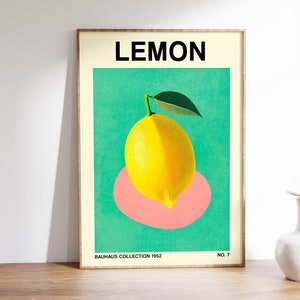The image showcases a photograph of a framed art print leaning against a white wall. The wooden surface beneath it appears to be a desk or table, also featuring a partially visible white vase on its right edge. The art print itself is centered and presents a striking, graphic depiction of a lemon. The lemon is bright yellow with a green leaf, sitting atop a pink circle, against a bright green or aqua background. Above the lemon, bold black letters spell out "LEMON," while the bottom of the print features the text "Bauhaus Collection 1952" on the left and "Number 7" on the right. The print is bordered by an off-white mat and encased in a thin, light wood-colored frame. The entire image is accentuated by light shading from the left, adding depth to the scene.